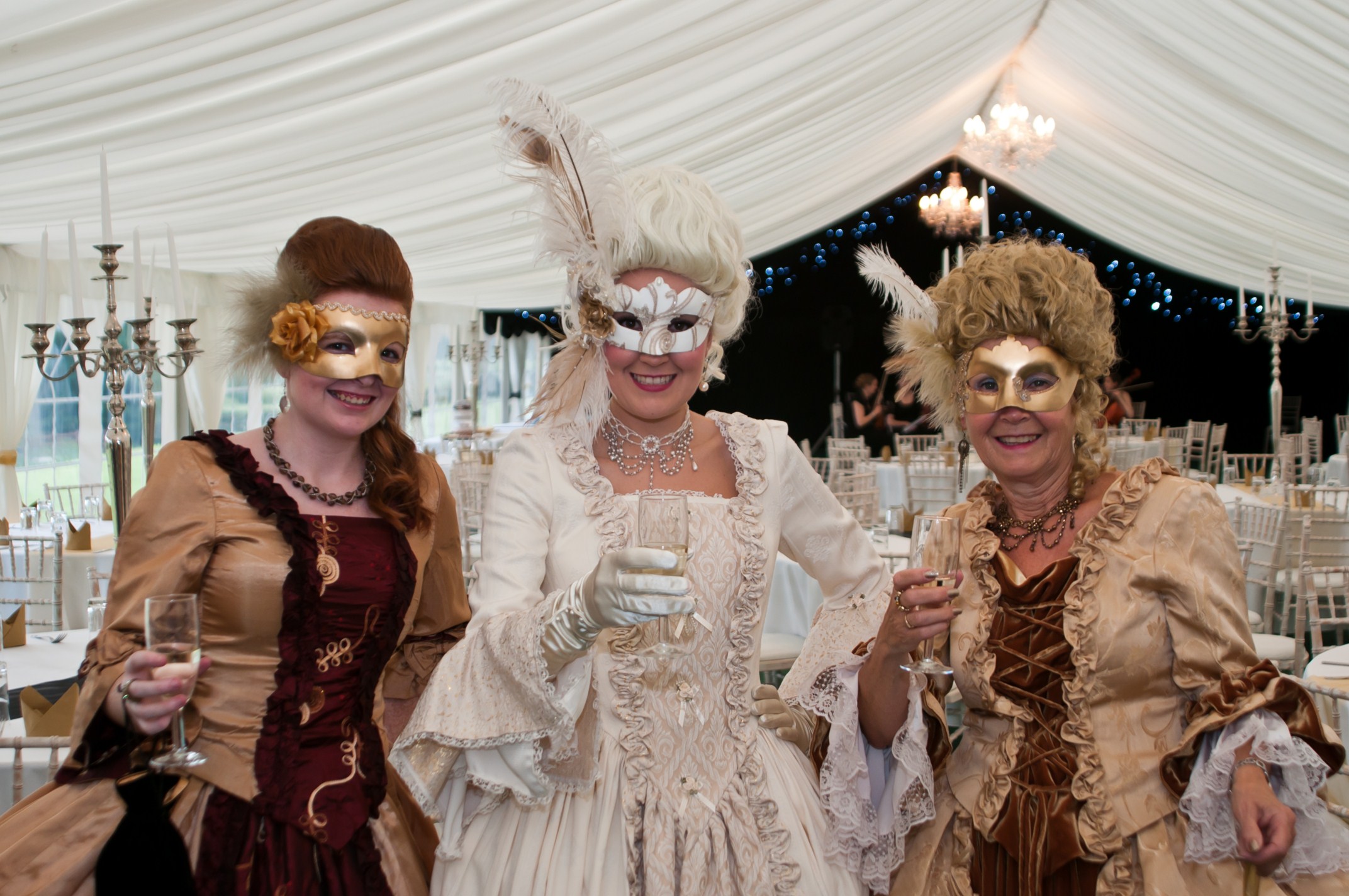In this detailed and photorealistic image, three women are dressed in masquerade masks and Victorian-era costumes, attending what appears to be a wedding reception set within an elegant, canopy-covered space. The setting, adorned with tall white drapes, elaborate tall candle holders, and chandeliers, features numerous ornate tables draped in white cloths and wood-braced chairs. 

Standing side-by-side, the woman on the left is wearing a light brown dress with a red flare covering her chest, holding a wine glass in her right hand. Her mask is gold. The woman in the middle, slightly older than the others with poofy white hair and a white mask adorned with a feather, is dressed in a white off-white blouse dress and wears a white glove on her right hand while holding a glass of champagne or wine. The woman on the right has light brown hair, a gold mask without feathers, and is dressed in a darker brown blouse with a brown material draped over her chest. Each woman is elegantly poised, contributing to the sophisticated and festive atmosphere of the masquerade-themed wedding reception.